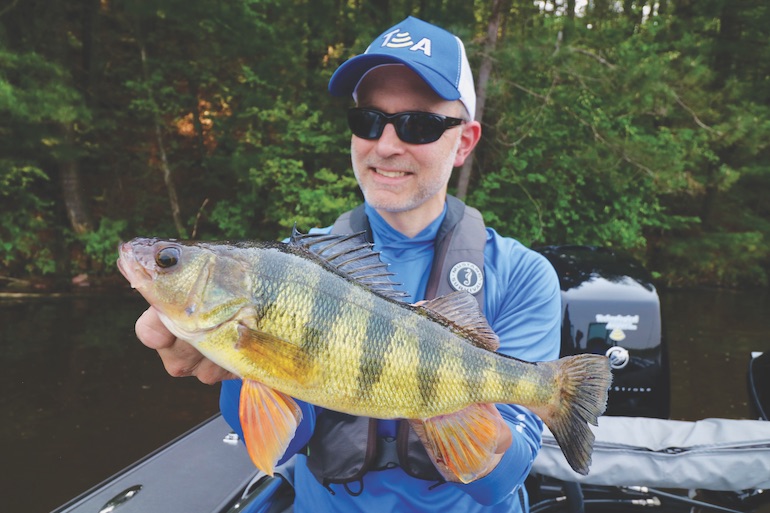A cheerful middle-aged fisherman, with gray stubble and wearing black sunglasses, proudly displays his sizable striped bass for the camera while seated in a gray motorized boat. He sports a blue long-sleeve shirt and a gray life jacket adorned with a distinctive blue and white pin featuring a logo inside a blue circle, resembling a seahorse. His blue and white hat, emblazoned with 'TA', shades his beaming face as he grips the fish, its head pointing left and tail right. The bass has a golden hue with greenish stripes and fins that are orangish-pink. In the backdrop, a dense, lush green bank surrounds the river or lake, creating a picturesque setting that reflects his joyful accomplishment. The boat's glossy black outboard motor is also visible, further adding to the scene’s authenticity and detail.